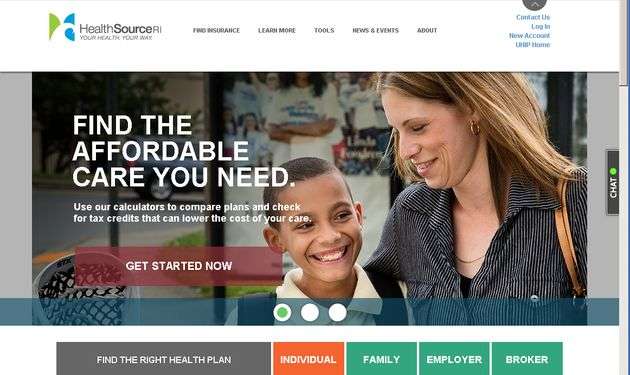The HealthSourceRI homepage prominently features the slogan "Your Health, Your Way" alongside a green and blue icon. The website is organized into various sections: Find Insurance, Learn More, Tools, News and Events, and About. Essential options such as Contact Us, Log In, and New Account are easily accessible.

Central to the page is a message encouraging users to "Find the Affordable Care You Need," highlighting tools for comparing plans and checking for tax credits to reduce care costs. A bold red button labeled "Get Started Now" prompts user action. 

The image features a woman in a suit shirt walking alongside a child with a backpack and collared shirt, set against an outdoor backdrop. A chat button with a green icon is available for instant assistance.

At the bottom of the page, tabs provide targeted information, labeled as Find the Right Health Plan, Individual with an orange background, Family, Employer, and Broker—with white text on green and orange backgrounds.

The clean, white background of the homepage is dotted with various buttons and navigational sections, offering a user-friendly experience to explore and learn more about health insurance options.